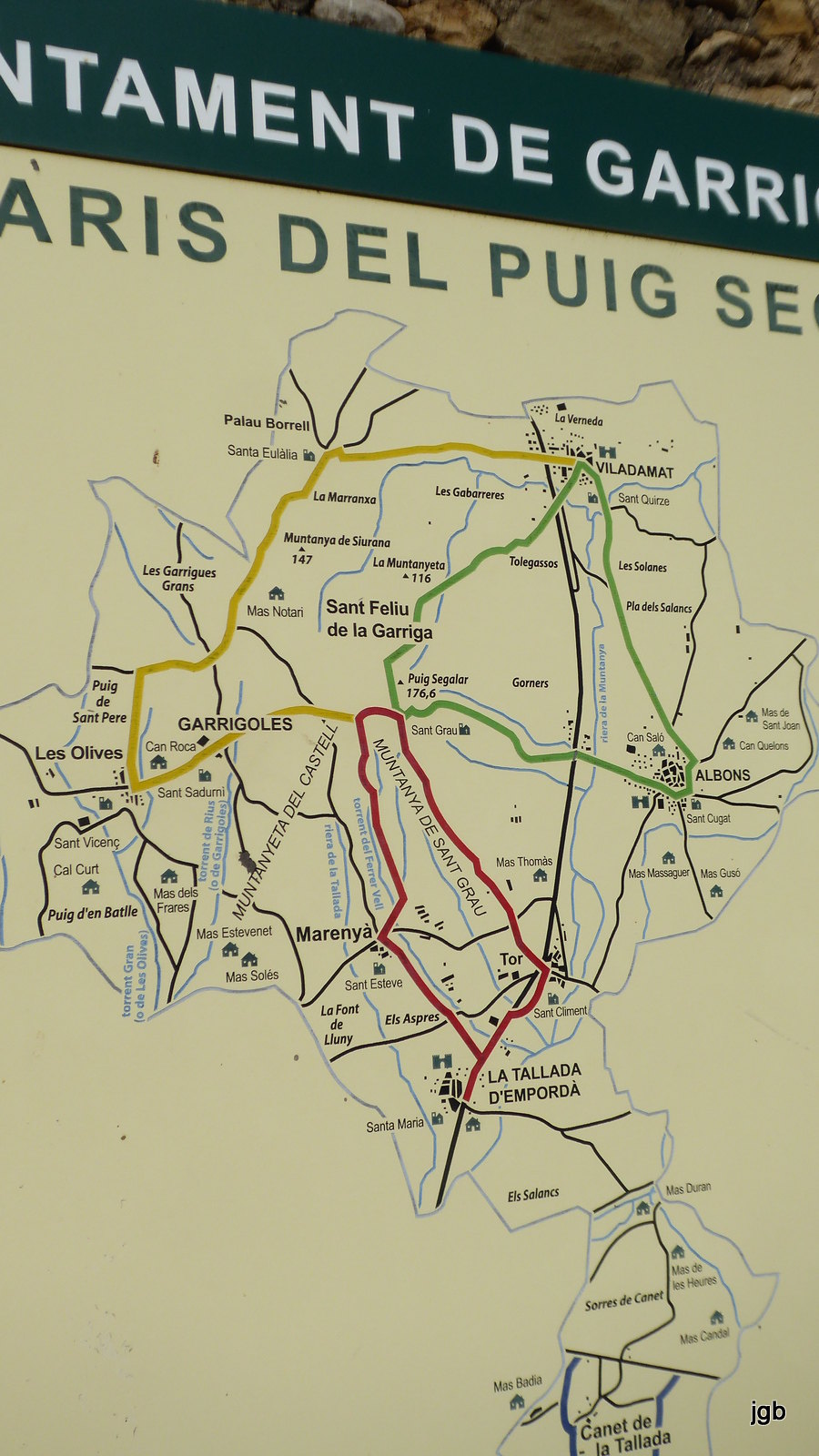The image depicts an intricately detailed map, possibly of a city, with indications of being Paris or another European location due to the French text. The map is adorned in multiple colors—yellow, green, red, and blue—delineating different regions or transit routes, including railways or bus lines. The titles and city names on the map are in French, with notable mentions such as "Albans," "Saint-Philippe de la Gare," and "Marigny et Montaigne de Saint Graal." Among the labeled points, a black strip with white letters spells "n-t-a-m-e-n-t-t-e-g-a-r-r-i," likely clipped from a larger word, and another section shows "A-R-I-S," suggestive of Paris, followed by "D-E-L," "P-U-I-G," and "S-E." The background of the map is primarily yellow and green, with white and black text denoting various locations. Notably, the top of the map features text in a green background with white lettering reading "Niamey-de-Garay" and another section with green lettering over a beige background stating "Arres-de-Puig-Sey." The map is rich in detail, presenting roads, rivers, and potentially small illustrations of buildings across towns, yet lacks any English text.